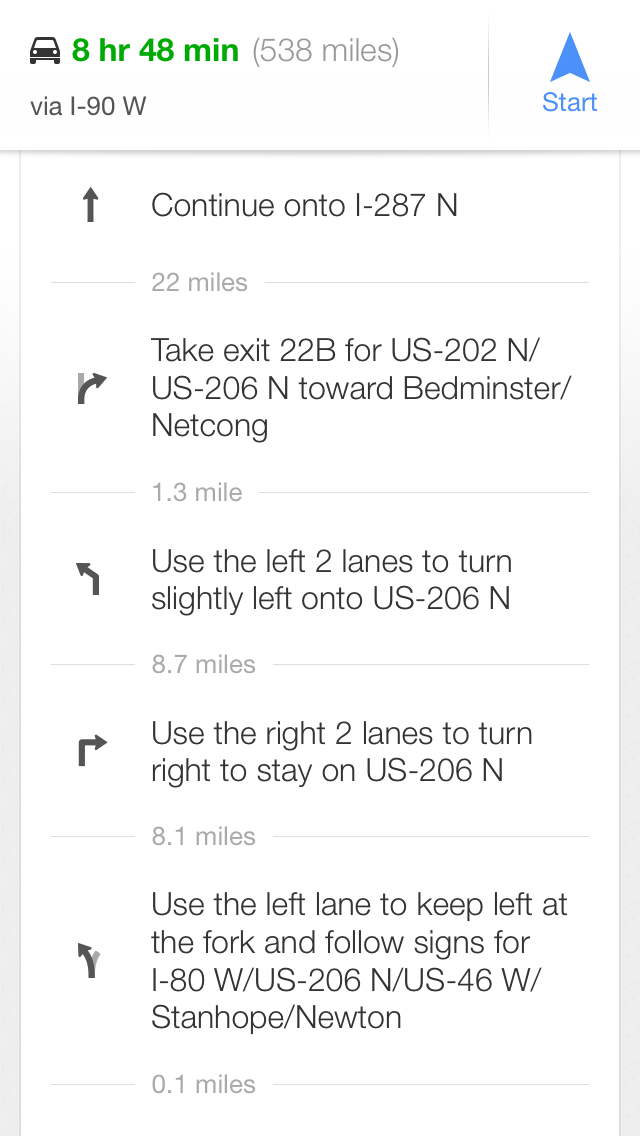The image is a screenshot from a smartphone showing GPS directions for an 8-hour and 48-minute car journey covering 538 miles via I-90 West. At the top left is a black silhouette of a car next to dark green text displaying "8 HR 48 MIN (538 miles)." Below, in black text, it reads "via I-90 W." On the right side, there's a dark blue triangle with the word "Start" underneath, indicating where to begin. The directions are detailed below:

1. Continue on I-287 North for 22 miles.
2. Take exit 22B for US-202 North / US-206 North toward Bedminster-Netcong and go 1.3 miles.
3. Use the left two lanes to turn slightly left onto US-206 North and continue for 8.7 miles.
4. Use the right two lanes to make a 90-degree right-hand turn to stay on US-206 North and drive for 8.1 miles.
5. Use the left lane to keep left at the fork, following signs for I-80 West / US-206 North / US-46 West toward Stanhope-Newton for 0.1 miles.

The directions are clearly laid out beneath these icons, guiding step-by-step through the journey.